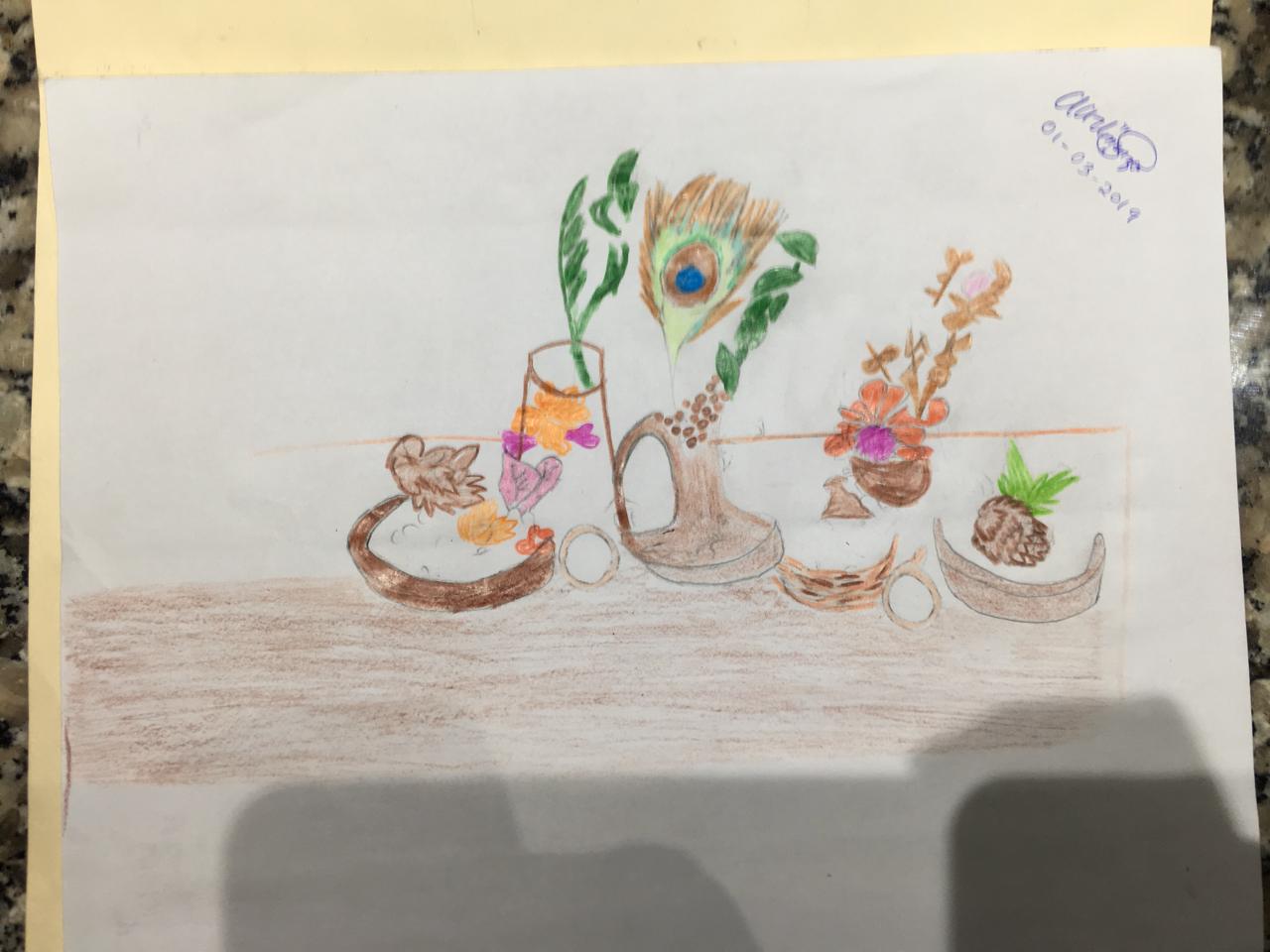In this vibrant color photograph, we see a carefully crafted drawing nestled in what appears to be a manila folder, with a hint of the folder visible at the top of the image. The artwork, likely created with colored pencils or pastels, exudes a whimsical charm. It features a simply drawn brown table, sketched in a rudimentary yet endearing style. On the table sits an intriguing assortment of items: a delicate peacock feather, a diminutive pineapple, and a small bowl brimming with orange and purple flowers. Additionally, there is a water glass adorned with intricate designs. The artist's signature graces the upper right-hand corner of the drawing, though it is indecipherable, but the date, "October 3rd, 2019," is clearly legible. This delightful visual composition captures a playful and imaginative snapshot of everyday objects.